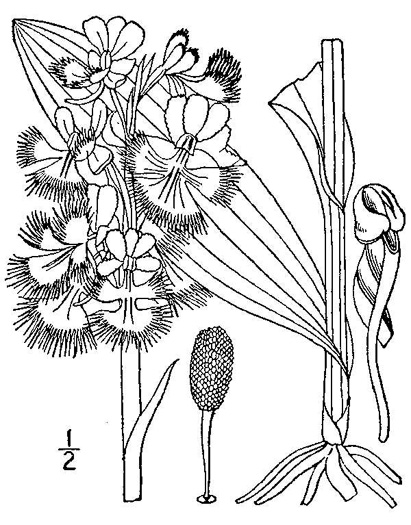The black and white marker drawing depicts a complex botanical scene with significant detail and variety in plant forms. On the left side, tall flowers emerge from the ground, their stems straight with a point splitting to the upper right. The flowers atop the stems have open buds adorned with long black hairs, transitioning to petals free of strings at the very top. A fraction, 1/2, is inscribed in the bottom left corner. Behind these flowers, a cob-like item wrapped in black lines and rounded at the top and bottom stands out. This cob is entangled at the base with what resembles a post or a pole, surrounded by finger-like structures extending into the ground. Further right, the drawing features an array of botanical elements, including leaves in a circular, upward-spiraling manner. This plant section, comparable to a mushroom on the verge of opening, features a white tube rising into a sock-like figure. Additionally, there's a tall pole with a multi-legged stand supporting it, reaching towards the top right and expanding leftwards. The right-most section contains what appears to be a chest, striped in black and white, possibly representing a figure without legs. The illustration encapsulates a rich mixture of flowers, stems, and an enigmatic structured form, all intricately intertwined and detailed.